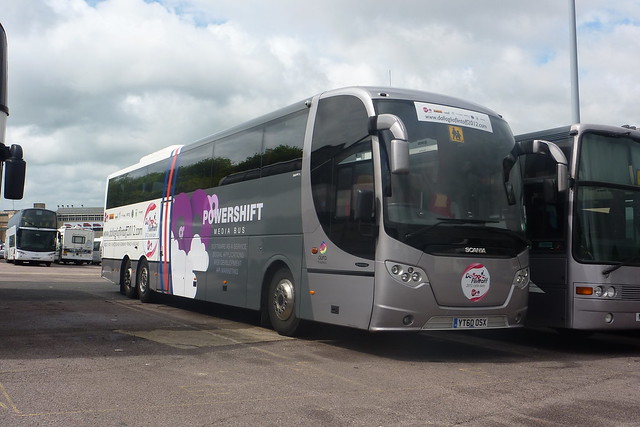This photograph captures a large parking lot filled with several buses. Dominating the scene are two large, identical gray buses parked closely side by side. The central focus is on a modern passenger bus bearing the inscription "Power Shift Media Hub" on its side, flanked by two blue stripes and one red stripe. The bus has a prominently large windshield, Europlates, and the license plate reads YT600SX. The make of the bus is Sonia. On the side and the back of the bus, there is some advertising, though much of it is illegible.

The parking lot is paved with typical road asphalt. The sky overhead is mostly cloudy with some blue showing through, and no sunshine peeking out. In the background, several other buses and the tops of distant buildings are visible. A lamppost can be seen on the right side, and just a sliver of another bus is noticeable on the far left edge of the image. The scene is set in daylight with a predominantly overcast sky.